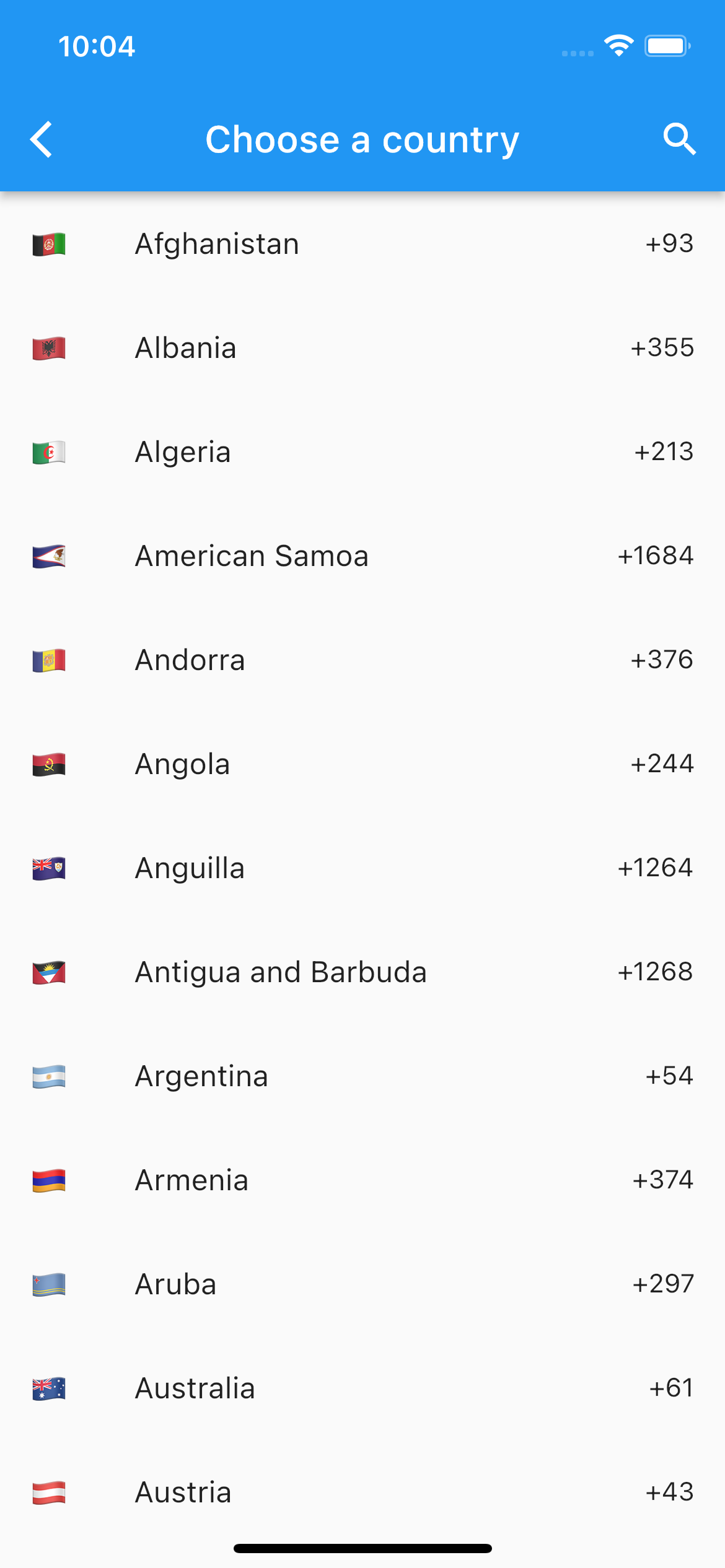On the screen, there is a prominent blue banner at the top with white text indicating "Choose a Country." To the right of this text, there is a small magnifying glass icon, presumably for search functionality, and to the left, there is a left-facing arrow for toggling back to the previous screen. Below the banner is a comprehensive list of various countries displayed with their corresponding national flags positioned to the left of each country name, which are slightly off-centered towards the middle of the screen.

The countries listed include:
- Afghanistan, with the country code +93
- Albania, with the country code +355
- Algeria, with the country code +213
- American Samoa, with the country code +1684
- Andorra, with the country code +376
- Angola, with the country code +244
- Anguilla, with the country code +1264
- Antigua and Barbuda, mistakenly merged as "Antigua, Mbarbuda" (should be separate as Antigua and Barbuda), with the country code +1268
- Argentina, with the country code +54
- Armenia, with the country code +374
- Aruba, with the country code +297
- Australia, with the country code +61
- Austria, with the country code +43

Each country name is accompanied by its respective international dialing code, providing a detailed overview useful for selecting a country based on its flag and dialing code.